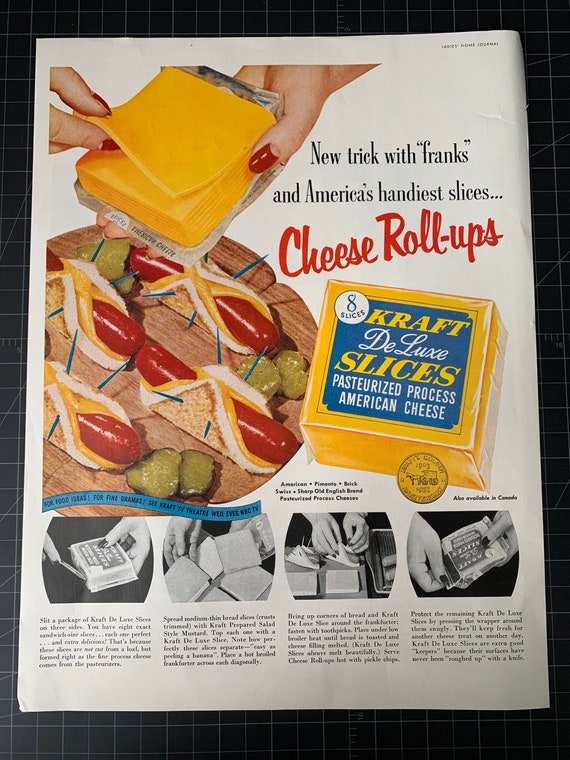The image depicts a vintage color-printed magazine advertisement for Kraft Deluxe Slices Cheese, displayed on a black gridded table. The white background of the ad accentuates its elements. In the top left corner, a photograph showcases a woman's hands peeling a slice of cheese from a package. Below this, on the left, there is a round wooden plate featuring reddish hot dogs wrapped in thin slices of bread, secured with toothpicks and melted cheese inside. Pickle slices accompany the roll-ups on the plate. To the right, in bold black text, it reads "New Trick with Franks and America's Handiest Slices," with "Cheese Roll-Ups" written in red, angled text beneath it.

The advertisement prominently features the Kraft Deluxe Slices packaging. The clear packaging reveals eight cheese slices, and the blue label on the front includes the following text: "Kraft" in yellow, "Deluxe" in white script, "Slices" in yellow block letters, and "Pasteurized Processed American Cheese" in white text. A gold seal is also visible on the packaging.

At the bottom of the ad, four black-and-white illustrations are displayed side by side, each with a small descriptive paragraph underneath. These illustrations depict the steps for preparing the cheese roll-ups: opening the package, placing cheese on a sandwich, wrapping the cheese-wrapped hot dogs with toothpicks, and sealing the cheese package. The overall design of the advertisement is clear and well-lit, showcasing a detailed and practical recipe for cheese roll-ups.